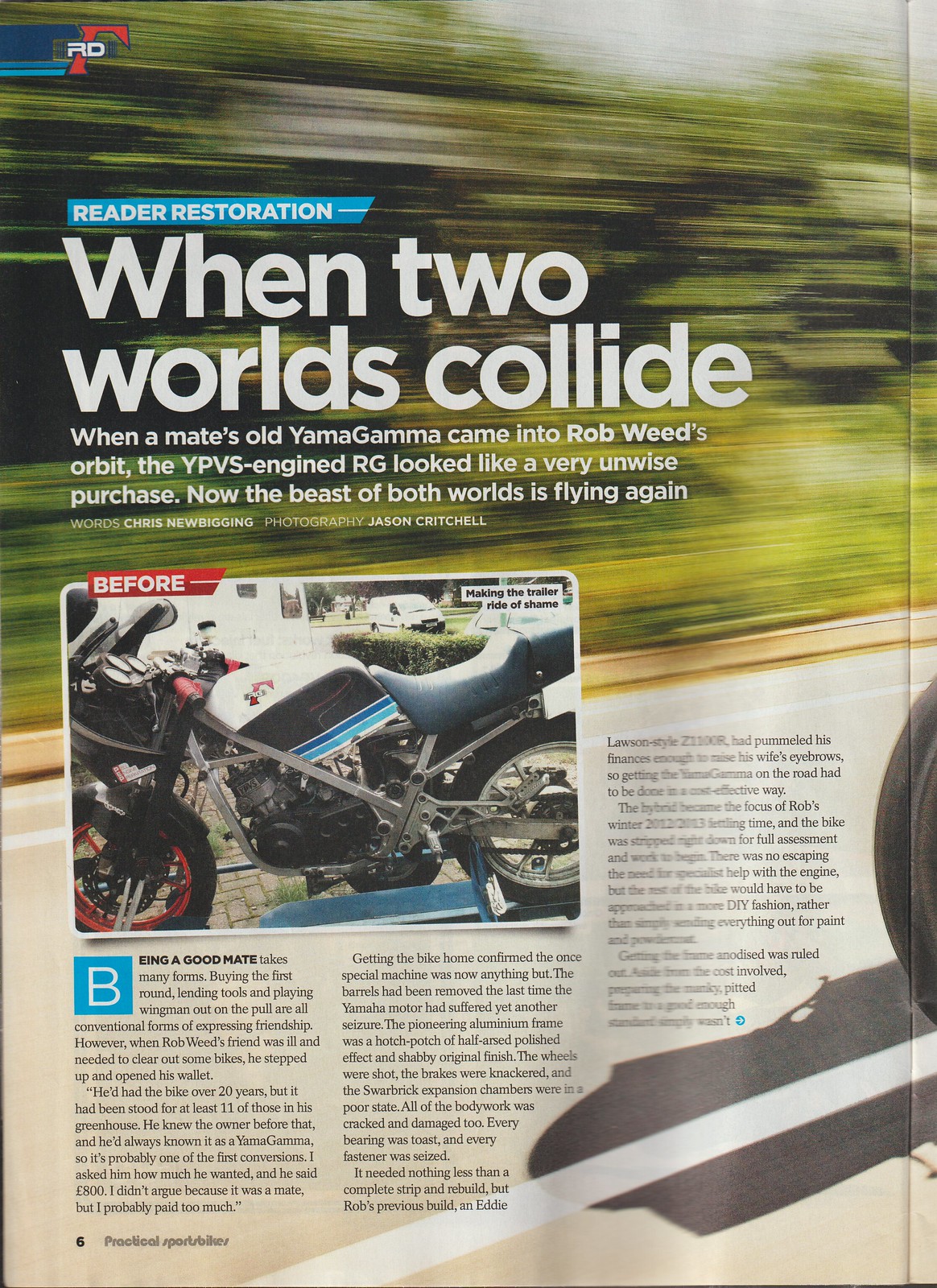This page from a motorcycling magazine, specifically page 6, features a reader restoration article titled "When Two Worlds Collide" in bold white block letters. The article highlights the story of a Yamagama motorcycle with a YPVS engine RG that initially seemed like an unwise purchase when it came into Rob Weed’s possession. However, through restoration, the motorcycle has been revived to combine the best of both worlds. The article's introduction, written by Chris Newbigging with photography by Jason Critchell, spans across three columns, indicating a detailed narrative of the restoration process. Featured prominently is a "before" picture of the bike, which is multicolored with black, light blue, medium blue, white, and red accents, captioned with "making the trailer ride of shame," hinting at its non-functional state at that time. The magazine is likely titled "Practical Sports Bikes," per the bottom of the page. The article suggests continuity beyond this page, delving into the comprehensive efforts involved in bringing the motorcycle back to life.